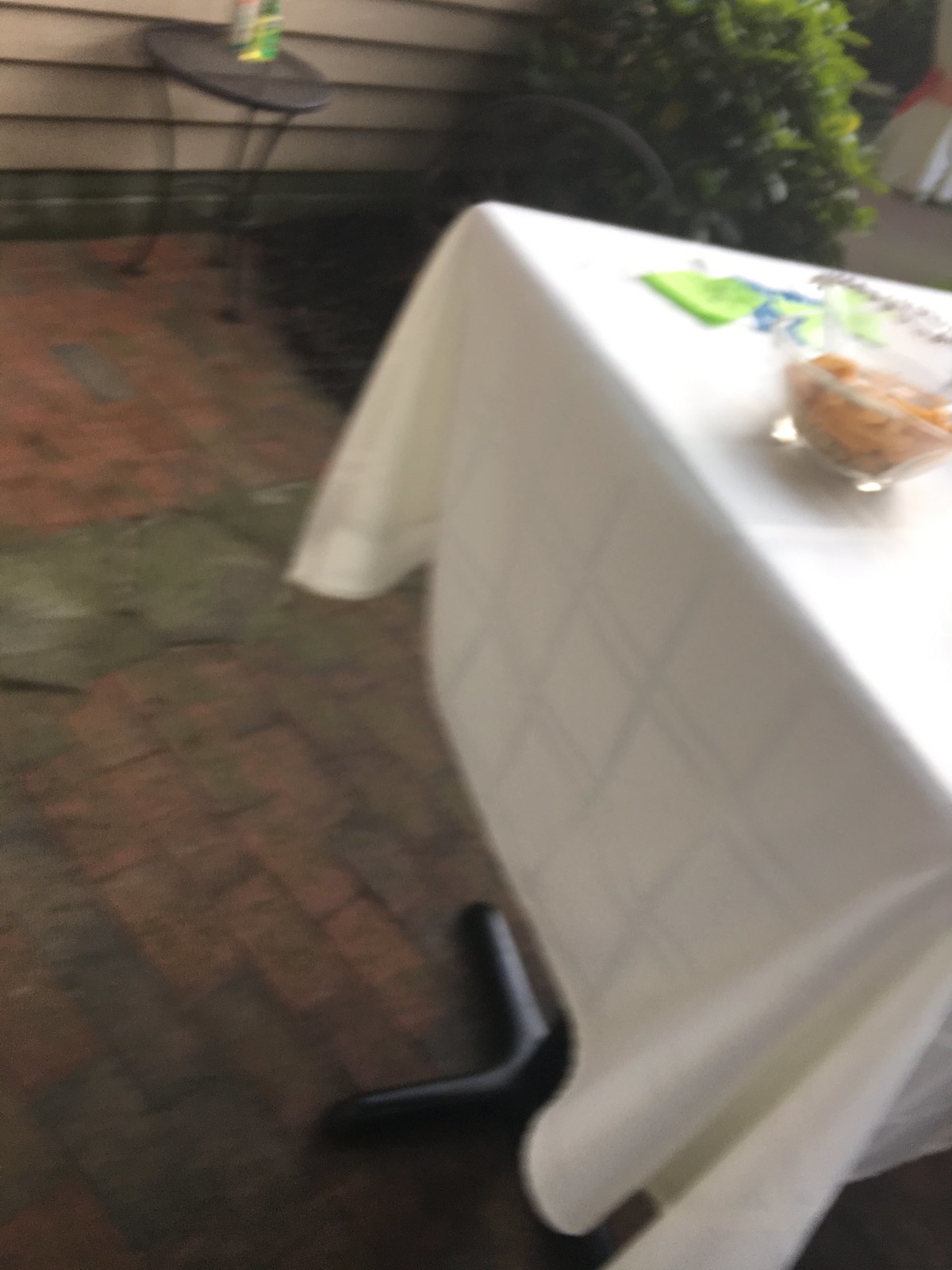A slanted outdoor photograph of a cozy patio area. The image captures a section of a patio with beige or brown house siding visible along the left side. In the foreground on the right side, a round, cast iron, three-legged patio table is partially draped with a white tablecloth. Atop the table sits a stainless steel bowl filled with light-colored items that resemble fortune cookies. A lime green napkin is casually placed near the bowl. The patio floor, made up of red bricks with patches of green moss, extends upwards at an angle due to the camera tilt, creating a dynamic perspective. In the upper right corner of the photo, a lush green hedge adds a touch of nature to the scene. The entire composition primarily shows the ground and lower elements of this quaint patio setting, emphasizing the earthy and inviting atmosphere.